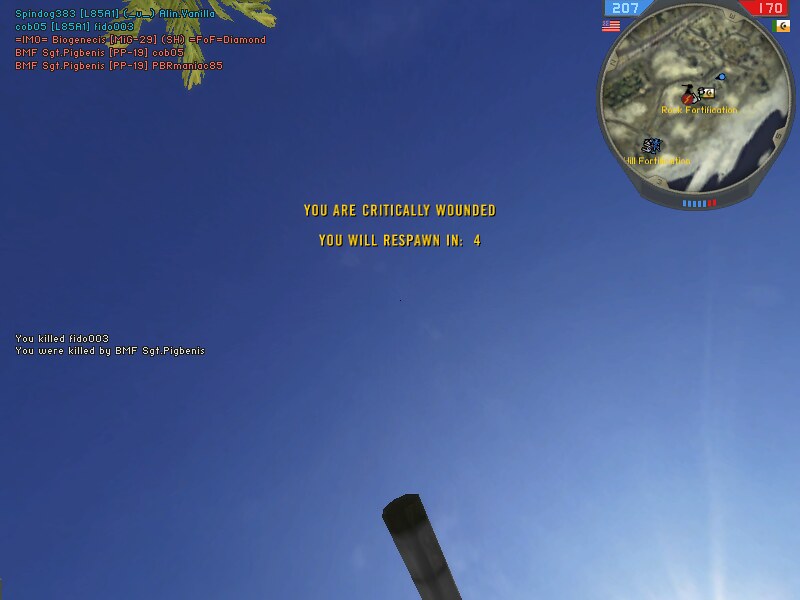The image is an in-game screenshot from a video game with a predominantly blue background, depicting a sky-like setting. In the upper right-hand corner, a circular, blurry map or compass is visible, accompanied by scores: 207 in blue and 170 in red. The top left corner displays names or stats, with text spanning five lines—the top two in blue and the bottom three in a reddish-salmon color. Central to the image, in yellow text, is the message "You are critically wounded," followed by "You will respawn in: 4." A notification in white at the left side of the image states, "You killed 50003," and beneath it, "You were killed by BMF Sergeant Peg Benes." Additionally, there's an image of a rifle or shotgun, emphasizing the first-person shooter aspect of the game. The setting also includes a palm tree in the upper left corner, adding to the detailed, immersive environment.